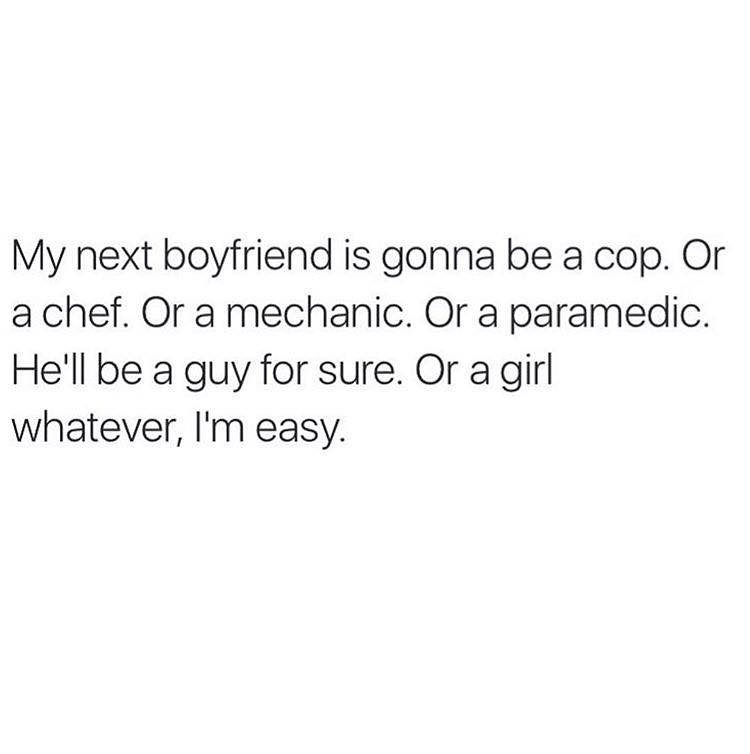The image features a plain white background with centered black text. The text is casual and straightforward, written in a small, thin, non-bold font, likely around size 14 or 16. It reads: "My next boyfriend is gonna be a cop. Or, a chef. Or, a mechanic. Or, a paramedic." On the next line, it states: "He'll be a guy for sure. Or, a girl. Whatever, I'm easy." The stark simplicity of the black and white, typewritten style suggests it might be a satirical meme intended for online sharing.